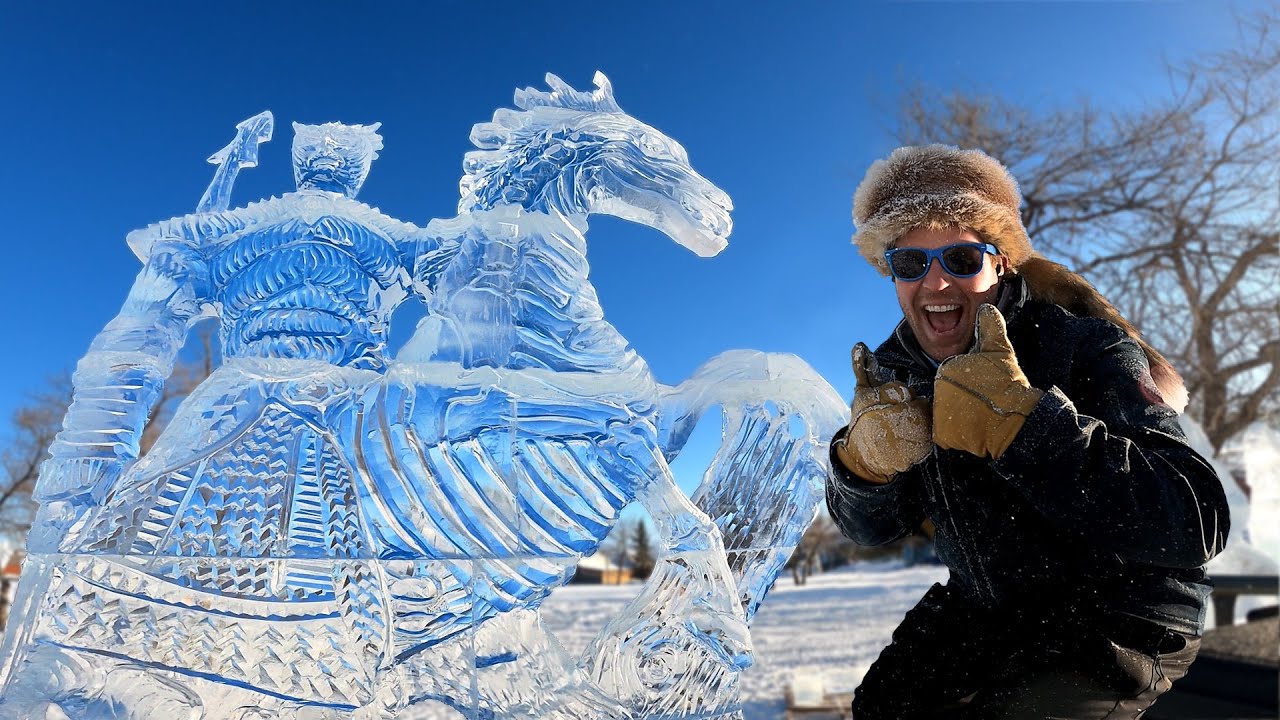In the image, a man is positioned on the right side, dressed in winter attire. He sports a raccoon-tailed fur hat, blue-framed sunglasses with black lenses, thick brown gloves, and an all-black or dark blue outfit. The man is smiling broadly with his mouth open, showcasing his top teeth, and he gives a thumbs-up gesture. Next to him stands a transparent ice sculpture depicting a heavily-armored person in motion, riding a horse and holding a sword in their right hand. The background features leafless brown trees, a clear blue sky, and a snowy ground. A gray structure, possibly a bridge, is faintly visible behind the sculpture, complementing the wintery outdoor scene.